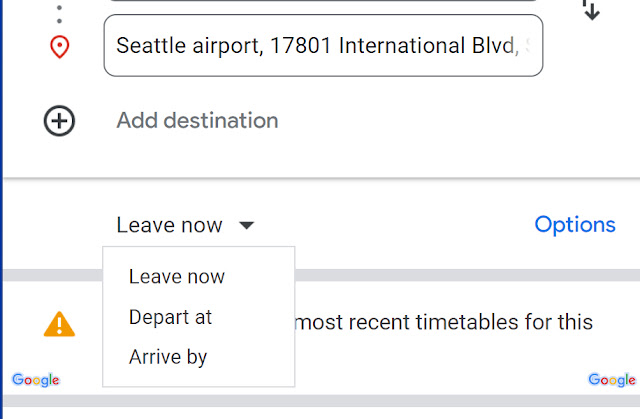A screenshot captures the lower section of an airport dispatch or trip planning page. Central to the image are two dots and a small red positioning icon, indicative of a map feature. The location is clearly marked as "Seattle Airport, 17801 International Boulevard." Beneath this, a circled plus sign invites users to add a destination, while a drop-down menu labeled "Contact" is actively selected. 

Further down, options for scheduling the trip are provided: "Leave now," "Depart at," and "Arrive by," each accompanied by a blue options tab and a settings button located to the right. In the bottom corners, Google's insignia is prominently displayed. There's also a partially visible yellow yield sign with a white exclamation mark, suggesting an alert or important notice. 

Finally, some contextual information appears to be truncated, mentioning "most recent timetables for this." Overall, the image likely depicts the lower interface of a flight planning or trip scheduling tool from Google, with various interactive elements and important travel details.